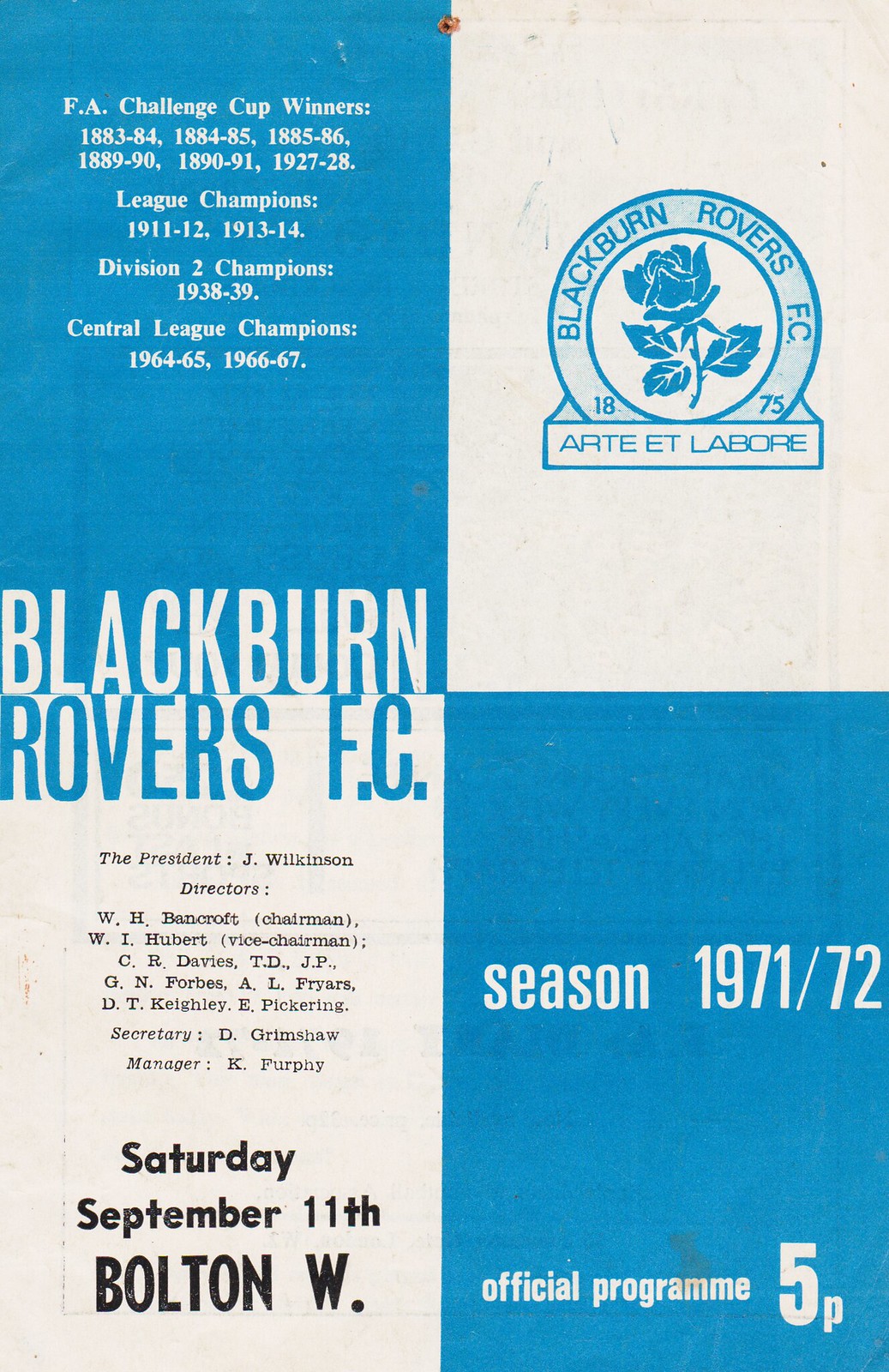The image depicts an old advertisement or program for a soccer game featuring Blackburn Rovers FC, dating to the 1971-1972 season. The layout is divided into four parts, alternating between blue and white rectangles with predominantly white and blue text. Key highlights include the club's logo—a blue rose encircled by the words "Blackburn Rovers FC 1875" and the motto "Arte et Labore" in the upper right corner. Additionally, it lists significant achievements in the upper left: FA Challenge Cup winners from 1883-1886, 1889-1891, and 1927-28, Division I champions in 1911-12 and 1913-14, Division II champions in 1938-39, and Central League champions in 1964-65 and 1966-67. The left side includes club details, mentioning key personnel such as President J. Rickinson, multiple directors, Chairman W.I. Hobart, Vice Chairman C.R. Davis, Manager K. Furphy, and Secretary D. Grimshaw. The program also indicates a match scheduled for Saturday, September 11th, against Bolton Wanderers, identified by "Bolton W." in black text. The notice specifies it as the official program, priced at five pence, for the season 1971-1972. The visual presentation of the card exudes a vintage aesthetic, characteristic of that era's sports advertising.